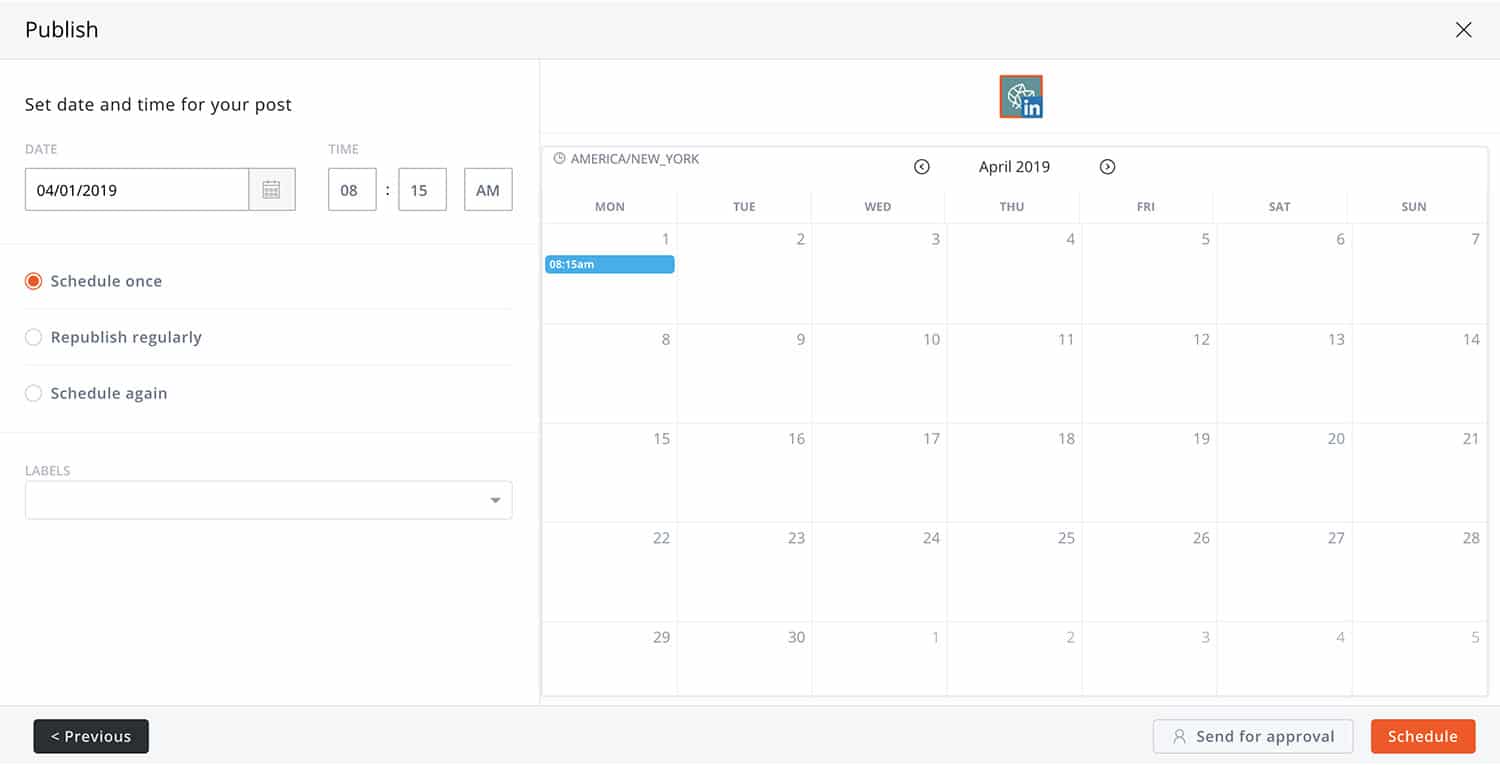The screenshot features a user interface for scheduling a post, set against a white background. At the top of the screen, a light gray horizontal banner spans the width, with the word "Publish" in black on the left and an "X" on the right.

Below the banner, on the left side, there's a section titled "Set Date and Time for Your Post," enclosed within a rectangle. The label "Date" appears a couple of lines down in gray, followed by a button displaying a date in black, accompanied by a calendar icon on the right, indicating that clicking it will open a calendar.

To the right, the label "Time" is positioned at the top, with three squares beneath it: the first showing "08", followed by a colon, the second displaying "15", and the third containing "A".

Further down, there are three option buttons outlined in gray. The first button, labeled "Schedule Once," is selected and highlighted in orange. The other two buttons are labeled "Republish Regularly" and "Schedule Again".

Below these options, there's a drop-down box titled "Label." On the right side of the screen, an extensive calendar for April 2019 dominates the space.

At the bottom left corner, there's a "Previous" button, which is a black rectangle with a white left arrow and the word "Previous" in white. On the right, two buttons are present: a white button labeled "Send for Approval" and an orange button labeled "Schedule" in white text.